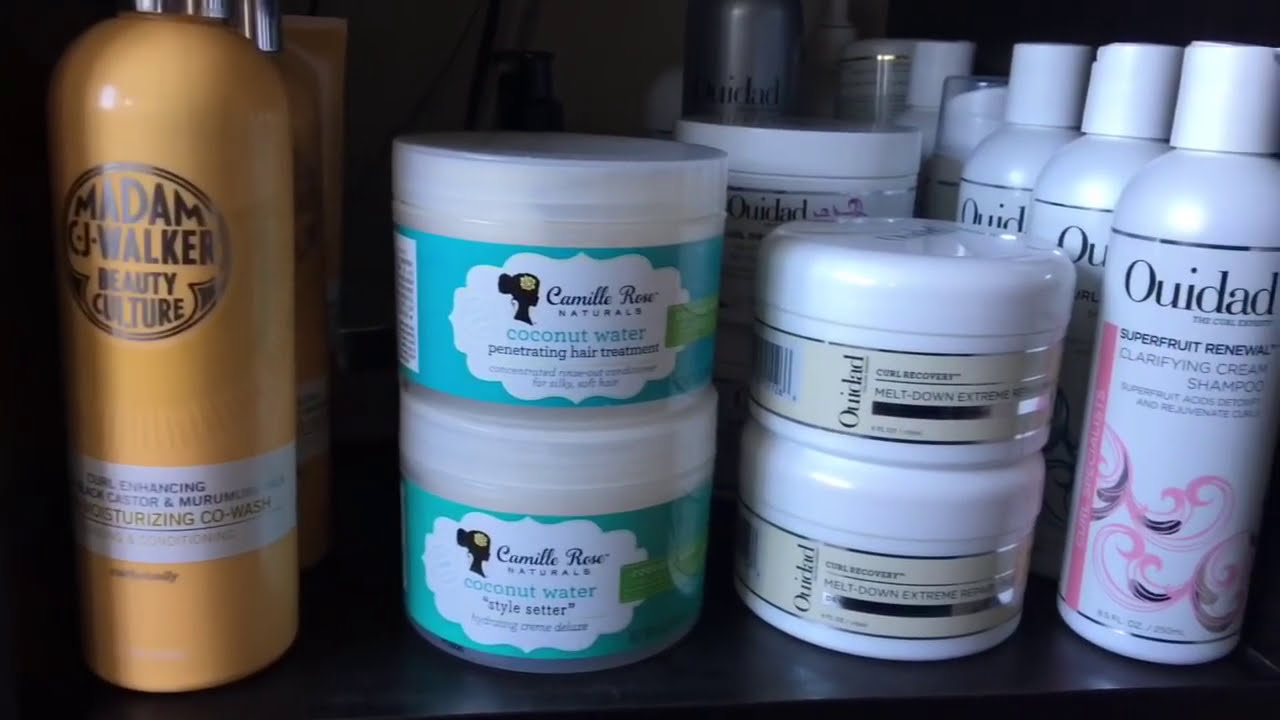This photograph captures a section of black shelving, likely in a salon or health and beauty aisle, displaying an array of hair care products. The shelves are filled with plastic bottles and containers, neatly aligned in both horizontal and vertical arrangements. The product lineup includes a tall, yellow bottle with a silver cap on the left, labeled "Madame C.J. Walker Beauty Culture Moisturizing Co-Wash" with a round logo in the middle. Moving towards the center, cylindrical jars of "Camille Rose Naturals Coconut Water Penetrating Hair Treatment" and "Camille Rose Coconut Water Style Setter" in beige and pink packaging stand out. To the right, another jar appears, branded with the name "Wee Dad Curl Recovery." The far right houses a slightly smaller bottle compared to the Madame C.J. Walker product, which is white with black and pink text, reading "Wee Dad Super Fruit Renewal Clarifying Cream Shampoo." The overall scene is brightly lit, with light reflecting off the plastic surfaces, emphasizing the vibrant colors of yellow, pink, beige, turquoise, black, and white. The setting suggests an indoor environment, focused on an organized display of beauty products.